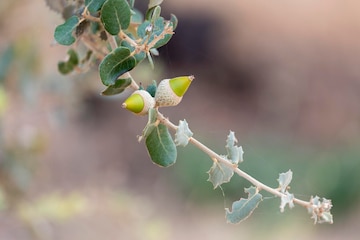A detailed close-up of a thin, light tan branch hangs diagonally from the top left to the bottom right of the image, captured in sharp focus against a backdrop that's completely blurred into a medley of cream, pink, green, and black hues. The branch is adorned with several oval-shaped leaves that display a gradient of green -- starting darker at the base and lightening as they extend outward. About midway along the branch's length, two unique, acorn-like structures with spiky bases protrude, featuring a white base and a green upper portion, resembling cone shapes with lime green triangular tops. The background outlines faintly suggest ground features and bushes, but they remain indistinct, enhancing the emphasis on the intricately detailed branch and its peculiar botanical elements in the foreground. No text or people are present in the image, bringing full focus to the natural beauty of the branch itself.